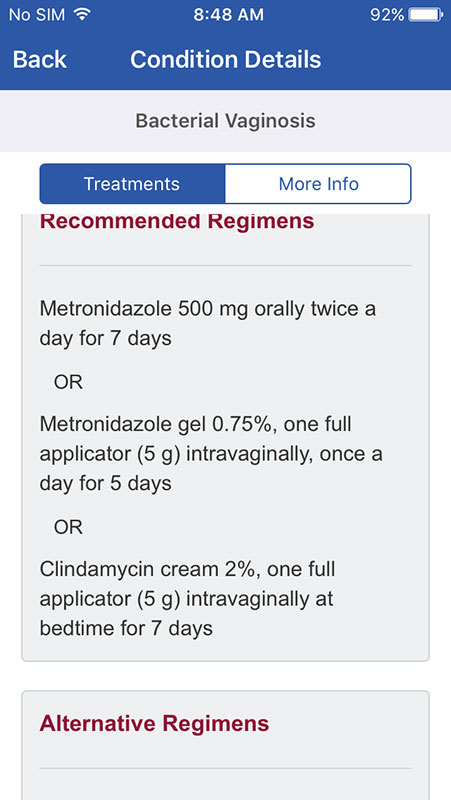Here is a detailed and cleaned-up caption for the image described:

---

The screenshot depicts a smartphone display at 8:48 AM, connected via Wi-Fi calling, with no SIM card installed and showing a battery level of 92%. The screen is displaying a page from a medical website, focusing on the condition details for Bacterial Vaginosis. The user has navigated to the "Treatments" section, which outlines recommended regimens for the condition. The treatments listed are:

1. Metronidazole 500 milligrams orally, twice a day for 7 days.
2. Metronidazole gel 0.75%, one full applicator (5 grams) intravaginally once a day for 5 days.
3. Clindamycin cream 2%, one full applicator (5 grams) intravaginally at bedtime for 7 days.

Additionally, options to view more information about the condition are available on the page.

---